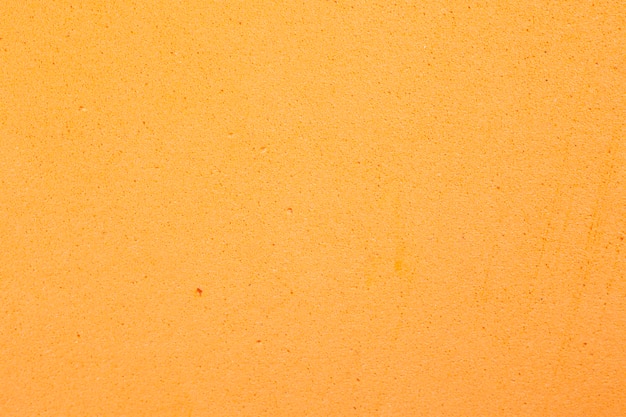The image depicts a textured surface resembling a manila envelope with its dull yellowish-orange coloration. It appears to be a firm, hard material, likely a wall made of concrete or possibly plaster. The surface is characterized by numerous small recessed holes, resembling pores or air bubbles found in volcanic rock. These holes are scattered across the surface, creating a pitted appearance. Additionally, faint horizontal streaks and scratches are visible, particularly more pronounced on the right-hand side, suggesting marks similar to those left by a car key or an animal's claw. The paint within the scratches appears slightly deeper gold. Overall, the image captures a plain orange-colored background with no additional patterns, text, or distinct features, just its natural textures and imperfections.